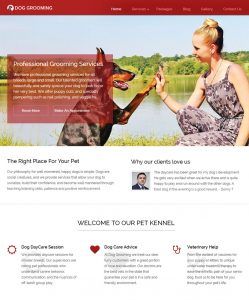The screenshot captures a visually appealing website dedicated to pet grooming services. At the top, a bold red text box featuring the phrase "DOG GROOMING" is prominently displayed in all caps with white text. 

Beneath this, there is a vibrant image showcasing a cheerful interaction between a woman and a Doberman. The woman, sporting a sleeveless floral top and matching floral pants adorned with dark purple and pink patterns, has her blonde hair styled in a bun and possesses a fair complexion. Positioned on the right side of the picture, she is engaged in a high-five with the Doberman, which stands on the left. The dog, predominantly black with light brown patches on its muzzle and paw, displays large, pointed ears.

This joyful scene unfolds against the picturesque backdrop of a lake with brownish water, surrounded by lush green trees and a clear blue sky overhead. 

Below the image, an organized section of text boxes is presented. The left box declares, "The Right Place for Your Pet," while the right box expresses, "Why Our Clients Love Us." Further down, additional information welcomes visitors to "Our Pet Kennel." The section continues with three well-defined columns, labeled "Our Daycare Sessions," "Dog Care Advice," and "Veterinarian." Each column contains smaller text brimming with detailed information, which, though somewhat difficult to read, suggests a comprehensive range of services offered by the establishment.